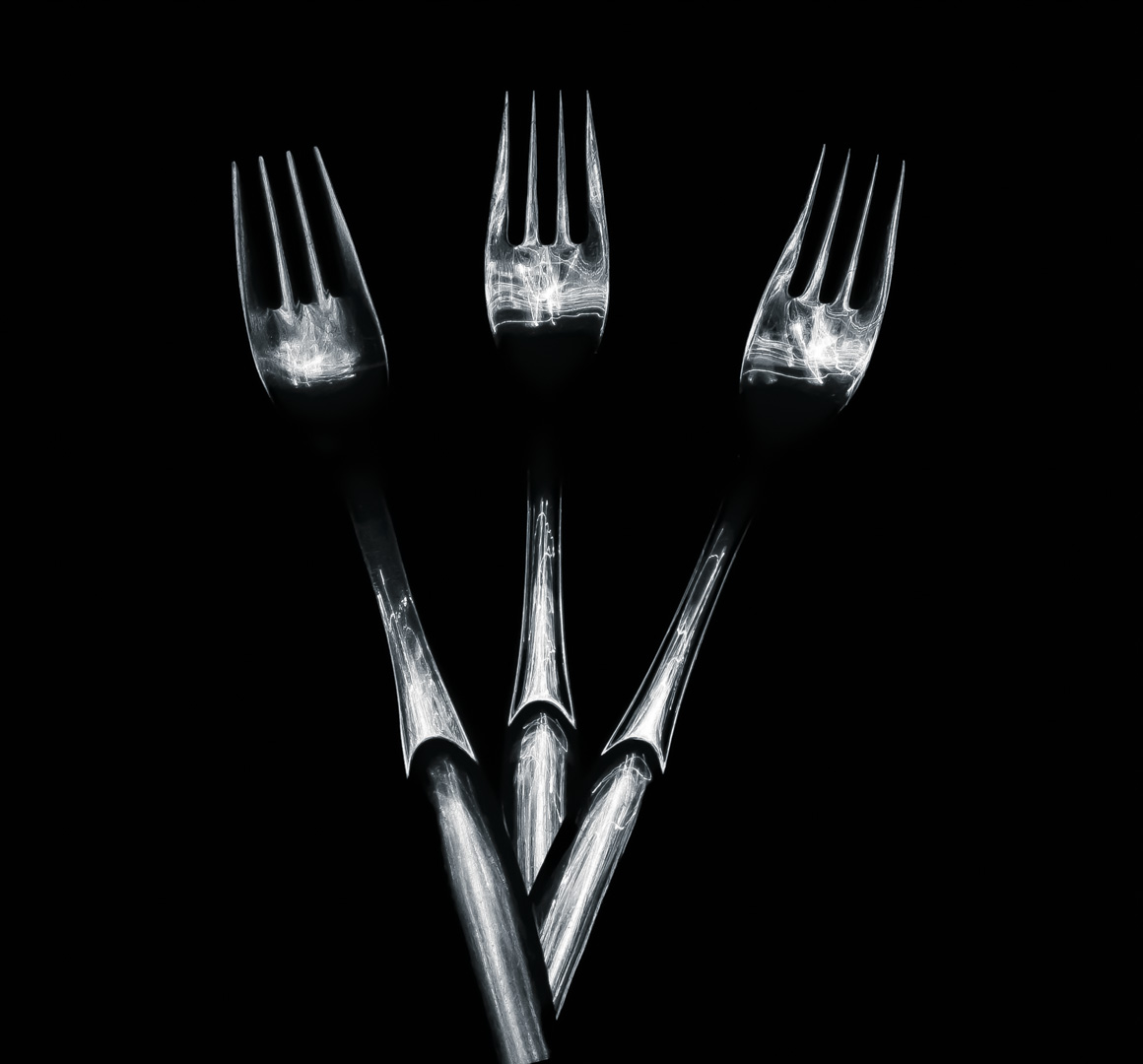The image depicts three silver-colored forks arranged in a crisscross fashion against a black background. The forks, angled and emerging from the bottom middle of the frame, are elegantly placed with their tines shimmering under the light. Each fork, standard in design, features four tines and a handle that subtly curves at the midpoint, becoming more slender as it approaches the pronged end. The central fork appears slightly taller than the flanking forks. The shine on the forks highlights their pristine condition, free from scratches, and a faint black shadow accentuates the spot where the tines meet the handle, adding depth to the composition.